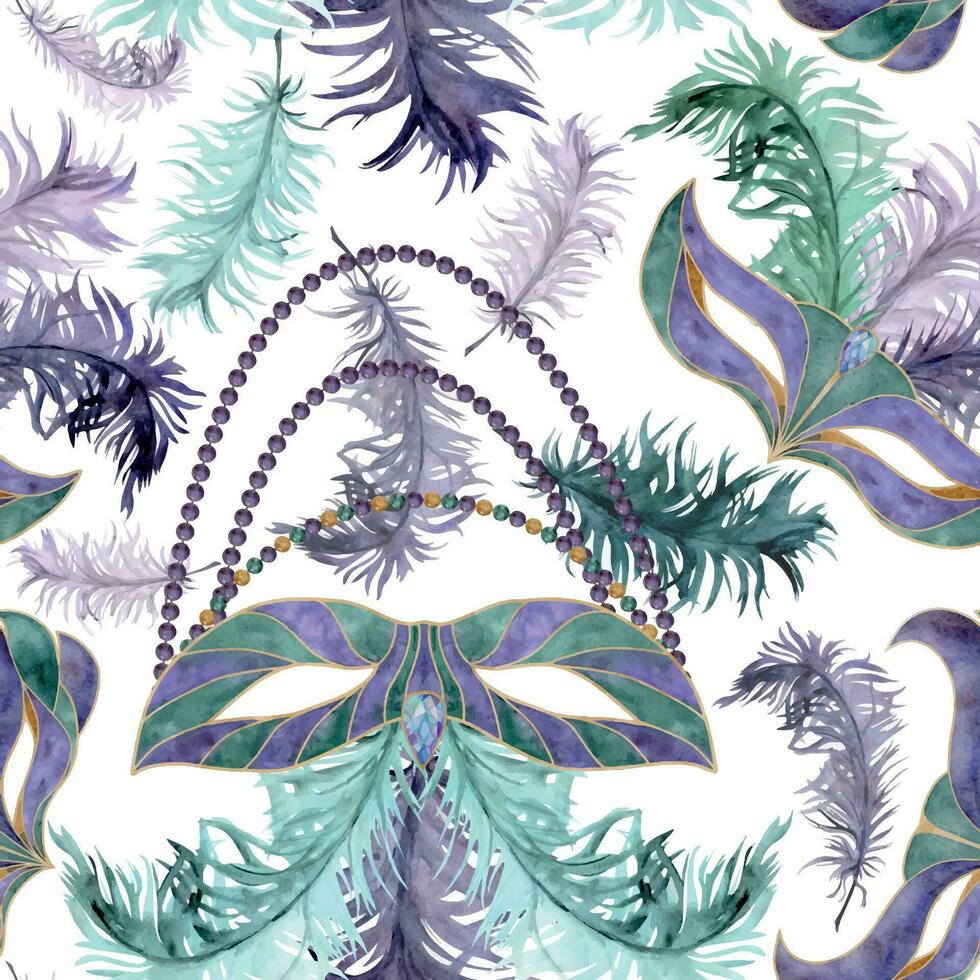This detailed illustration depicts an array of vibrant Mardi Gras masks adorned with colorful feathers and beads, sprawling across a white background. The masks, vividly painted in shades of blue, purple, green, and touches of orangey-brown and gold, create a festive atmosphere typical of a Mardi Gras celebration. Among the masks, two are prominently displayed while three others are partially visible, each contributing to the dynamic composition. One mask, positioned toward the lower center, features three strands of beads—two purple and one multicolored—dangling elegantly. Another mask, situated diagonally toward the top, boasts a small gem at its peak. Feathers in matching festive colors sprout from the masks and seem to float across the canvas, adding to the scene's sense of movement and celebration. The intricate patterns and scattered placement of the masks and feathers emphasize the lively and chaotic spirit of Mardi Gras.